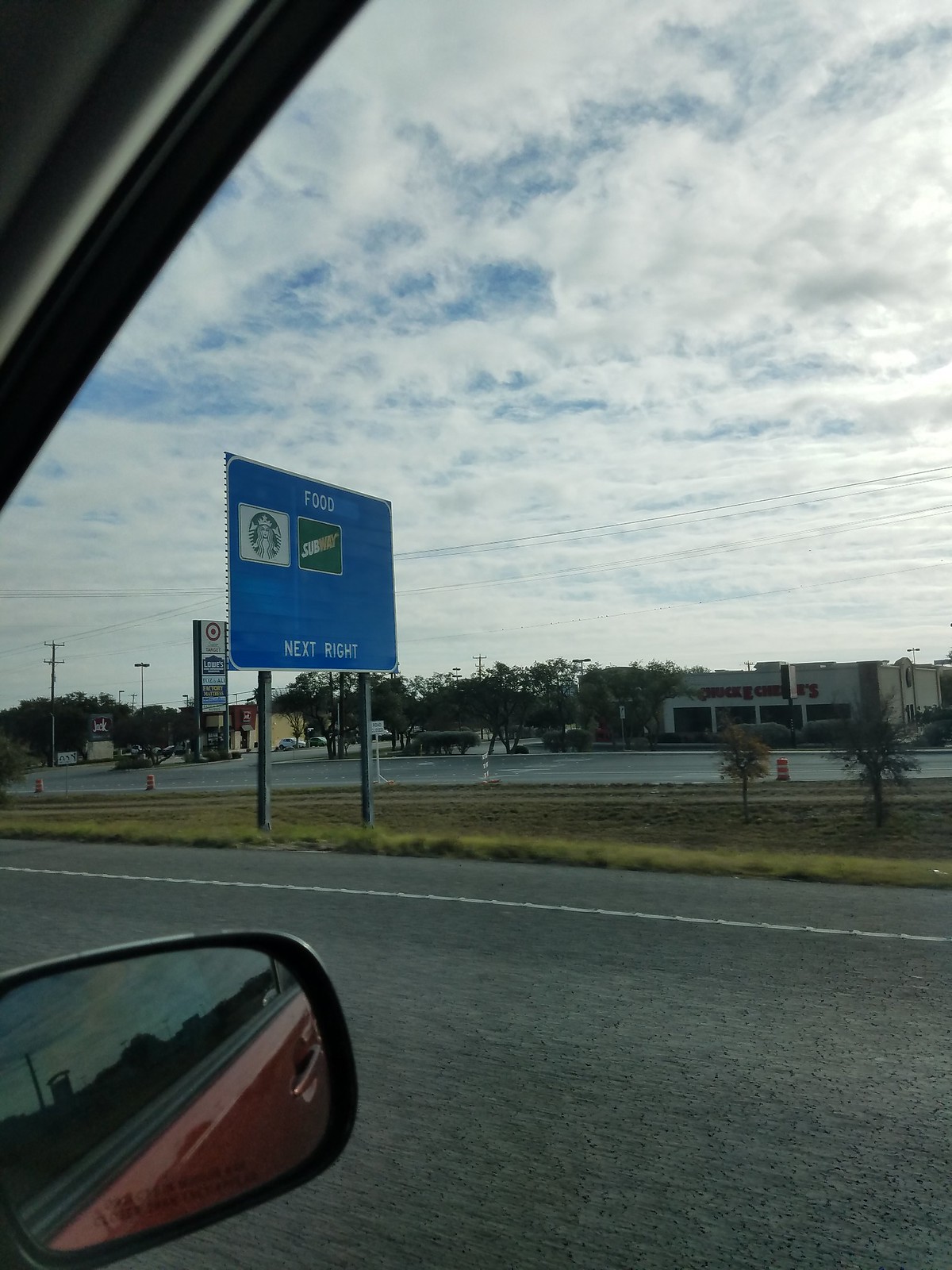This photograph, captured from within a vehicle, frames a highway scene through the vantage point of a side window. In the bottom left corner, part of the car’s side mirror is visible, reflecting a glimpse of the vehicle's red exterior. The upper left corner reveals a portion of the window frame, adding context to the car's interior perspective. The focal point of the image is a prominent blue rectangular highway sign, supported by two metal posts. The sign features white text at the top that reads "Food" accompanied by the iconic logos of Starbucks and Subway in two small rectangular boxes. Below, it directs drivers with the message "Next Right" also in white lettering. In the background, various buildings and additional signage can be seen, including one notable sign displaying the Target logo, contributing to the commercial atmosphere of the area.